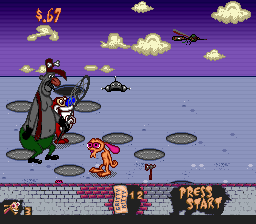This vibrant and colorful screenshot from an older, cartoonish video game captures a whimsical scene under a purple sky dotted with white, vanilla-colored clouds. At the top left corner, the balance shows 67 cents. The ground below is a striking blue, interspersed with grayish-maroon walls. In the lower right-hand corner, a black box with gold letters prompts players to "Press Start," while the text "Gritty Kitty" is visible at the very bottom.

The scene showcases three distinct characters. The first is a short, orange character with pink eyes and ears, likely a rabbit. The second character, described as a large, gray person with a prominent nose, is holding a smaller figure who has a blue nose and wields a net, smiling at the presence of a fly above. This smaller figure is dressed in green pants with red suspenders and a hat, resembling a bird with an enormous orange beak. Lastly, a maroon-colored cat with a white face rounds out this eclectic group. Each character adds to the playful and imaginative atmosphere of the game.